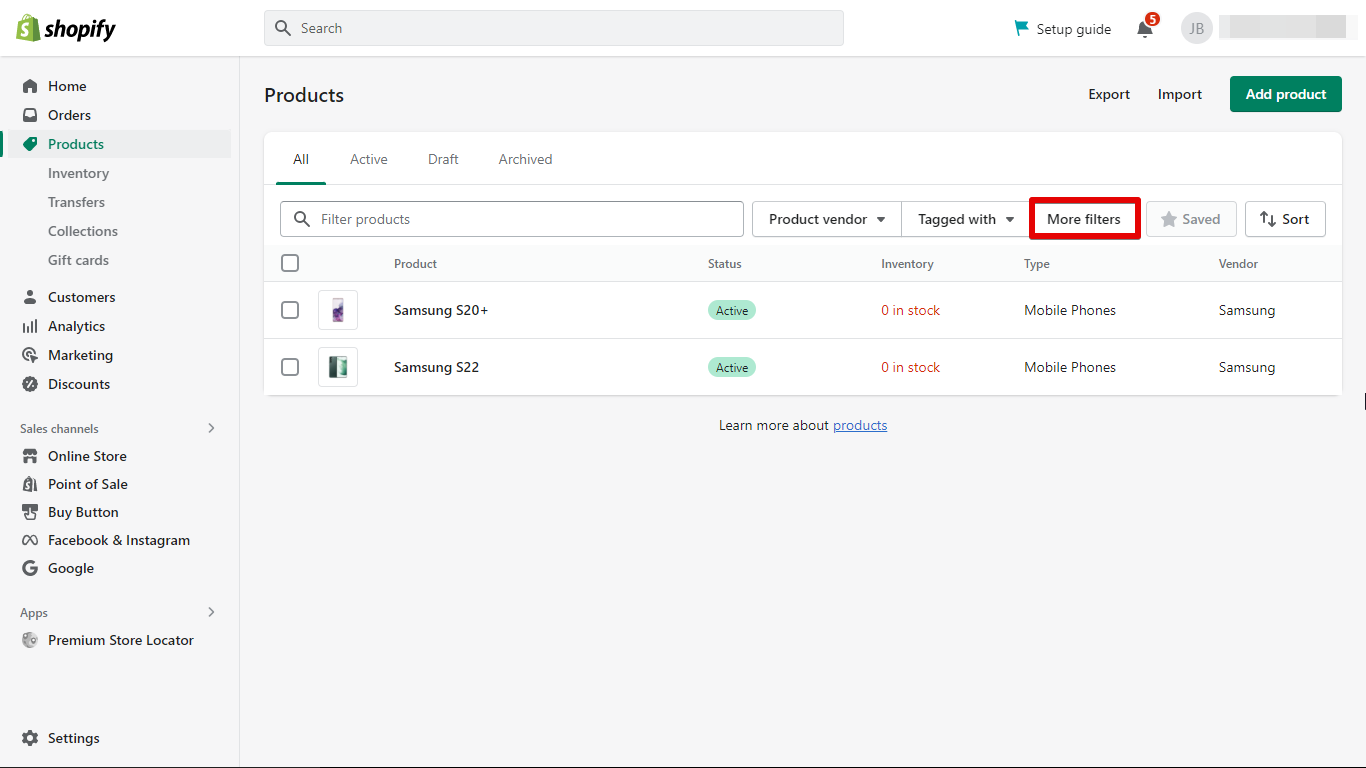An image captures a detailed view of a Shopify admin panel, showcasing a user's cart page. The interface features a predominantly light blue background. Along the left-hand vertical sidebar, the Shopify logo is prominently displayed, represented by a green shopping bag with a white "S" in the center. Below the logo, the menu items are listed: Home, Orders, Products (highlighted in green), Inventory, Transfers, Collection, and Gift Cards, all in light gray. Further down the sidebar are additional menu items: Customers, Analytics, Marketing, Discounts, Sales Channels, Online Store, Point of Sale, Buy Button, Facebook and Instagram, Google, Apps, Premium Store Locator, and Settings.

The top of the page includes a search bar, a setup guide marked by a small bluish flag, a notification bell with a red badge displaying the number 5, a gray circle with the initials "JB" inside, and a horizontal rectangular gray area. Below this header, the navigation options for Products are displayed: Export, Import, and Add Product (highlighted in a green box).

On a white background, the tabs All (underlined in green), Active, Draft, and Archive are visible, with “All” being the active tab. Below this, the product listings are detailed:

1. **Samsung S20 Plus**:
   - Thumbnail: Small purple image of the phone.
   - Status: Active.
   - Inventory: 0 (highlighted in red).
   - Type: Mobile Phone.
   - Vendor: Samsung.
   - Above "Type," a box labeled "More Filters" is outlined in red.

2. **Samsung S22**:
   - Thumbnail: Small image of the Samsung S22.
   - Status: Active (displayed within a small blue oval).
   - Inventory: 0 (highlighted in red).
   - Type: Mobile Phones.
   - Vendor: Samsung.

At the bottom of the product list, a blue underlined link reads "Learn More About Products." The image clearly shows this information with no additional text or images.